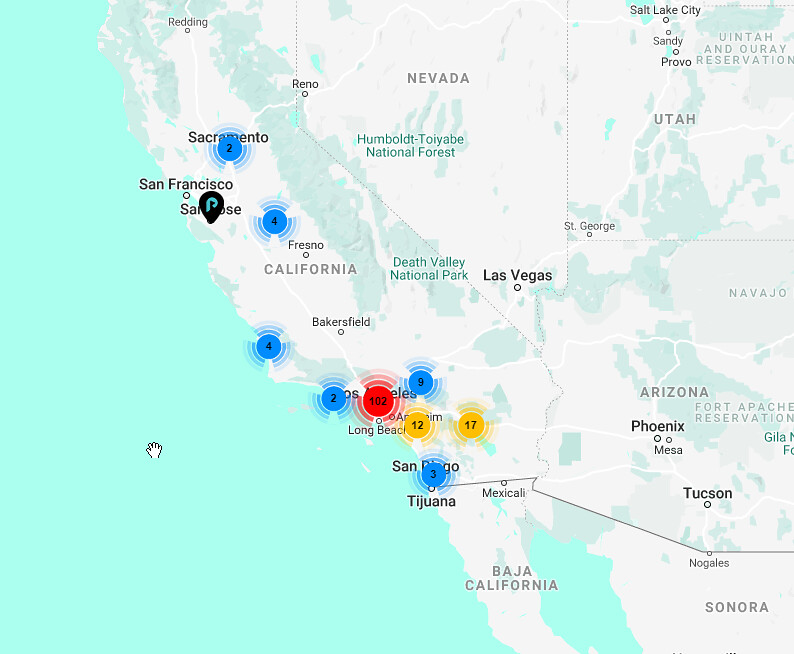This detailed regional map highlights the states of California, Nevada, Utah, Arizona, and Baja California. The primary focus is on various major cities within California, marked prominently across the map. Topographically, the map employs a color-coded scheme with gray representing general land regions and green signifying either forested areas or parks, though the exact nature of these green areas is unspecified.

Distinctive color-coded circles with numbers are dispersed throughout the map, indicating different points of interest or data sets. These circles come in blue, yellow, and red hues, each with radiating lines and numbers at the center. Smaller blue circles feature smaller numbers such as 2, 4, and 9. Yellow circles denote intermediate numbers like 12 and 17. A singular prominent red circle displays a significantly larger number, 102.

Key numbered points include:
- A blue circle with the number 2 over Sacramento.
- Two blue circles with the number 4 near Fresno and to the left of Bakersfield.
- Several circles, including yellow and blue, scattered around the Los Angeles region displaying numbers 2, 9, 12, and 17.
- A red circle with the number 102 positioned over Los Angeles and north of Long Beach.
- In the San Diego area, blue circles numbered 2, 3, and 9 appear.

There’s also a distinct logo over San Jose that is not recognized, along with a cursor in the form of a hand placed to the left of the visual. This suggests an interactive element to the map.

The exact significance of the numbered circles remains ambiguous, but they might represent data such as earthquake occurrences, crime rates, or another form of regional statistics.